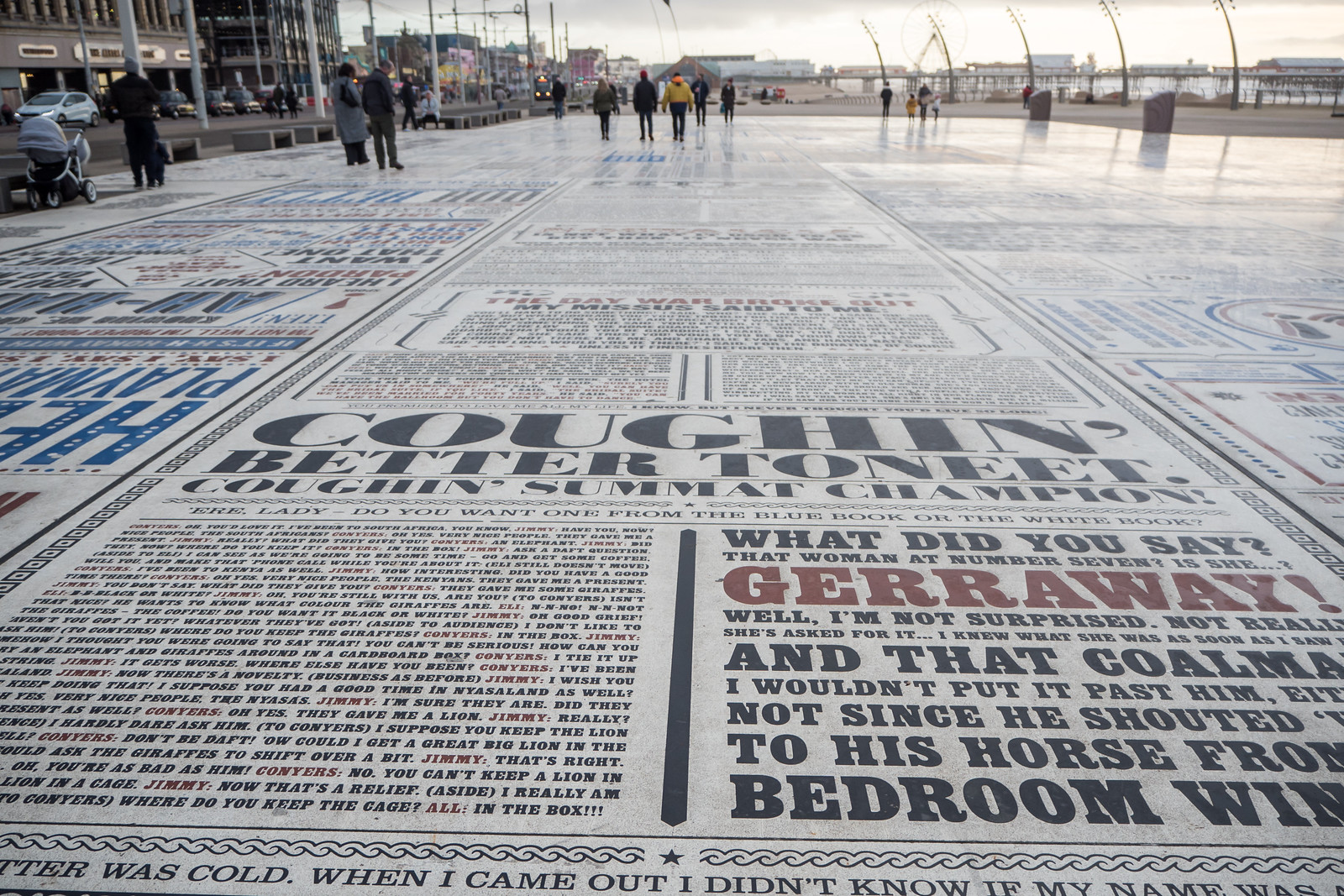The image displays a large outdoor plaza resembling a massive newspaper, with text of varying sizes scattered across the ground. People are walking and reading the text beneath their feet. A notable quote reads, "What did you say? What woman at number seven is she? Get away." Another prominent phrase includes "coffin, better to meet." On the left side, a man in a black jacket and pants stands by a gray baby stroller. Close to him, a woman in a gray jacket with a handbag over her right shoulder, accompanied by a man in a dark shirt and greenish pants, is also engrossed in the ground's writings. Stone benches are visible nearby, and the background reveals several cars, tall buildings, and signs, all under an overcast sky. The scene includes a mix of large black, red, and blue letters amid a plethora of smaller text, making the plaza's surface look intricately decorated as if covered by an immense, detailed newspaper.